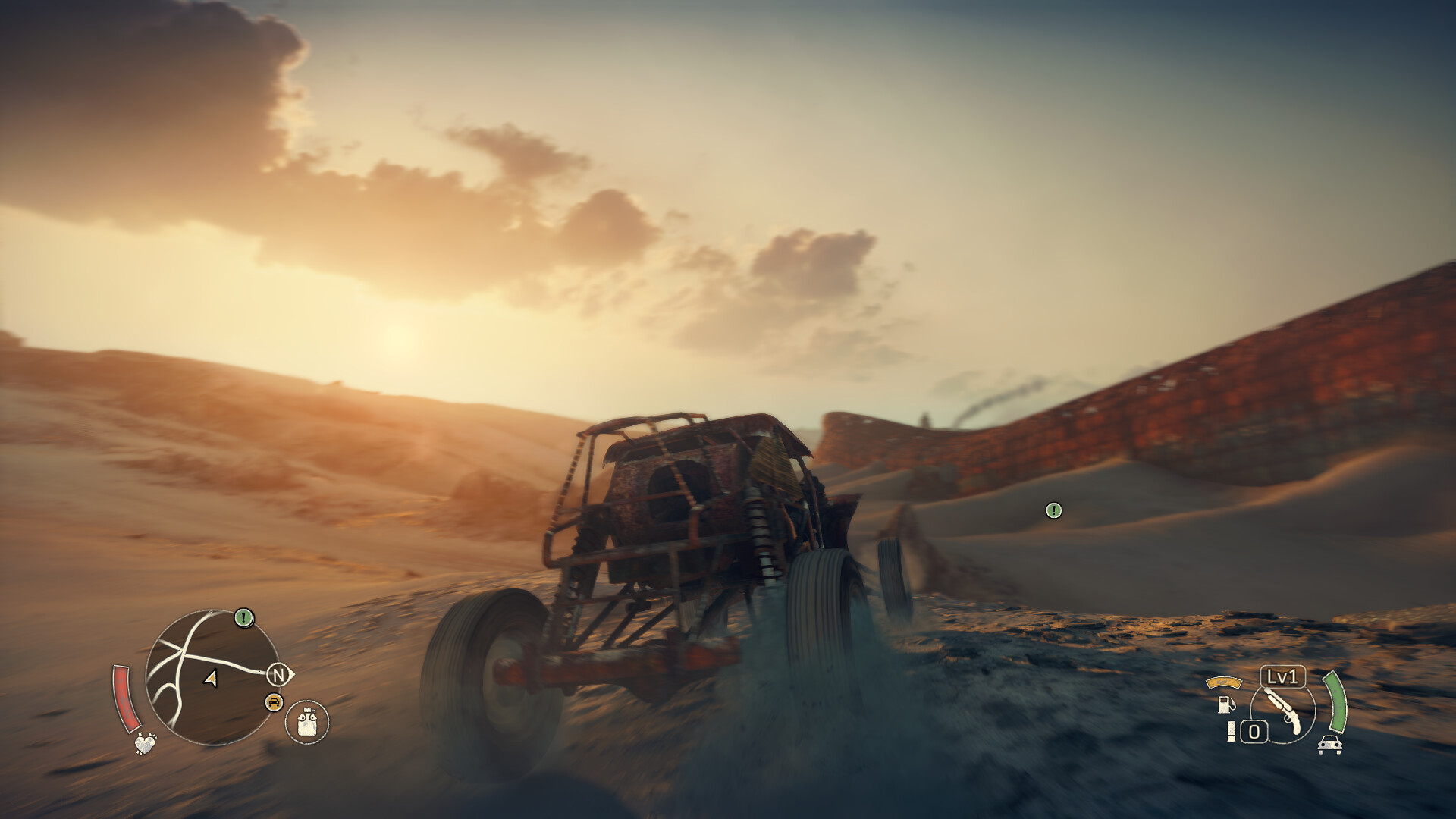The photograph captures a black dune buggy traversing the vast desert landscape, viewed from behind. The buggy, equipped with the typical protective metal bars and featuring a striking red rear axle, is seen heading towards a prominent red rock face or small cliff in the foreground. Surrounding the buggy, undulating dunes create a picturesque scene, with a particularly large dune that resembles a hill dominating the background. The expansive sky above is mostly illuminated by the sun, with a solitary wisp of dark cloud stretching across it, adding a touch of contrast and drama to the image.